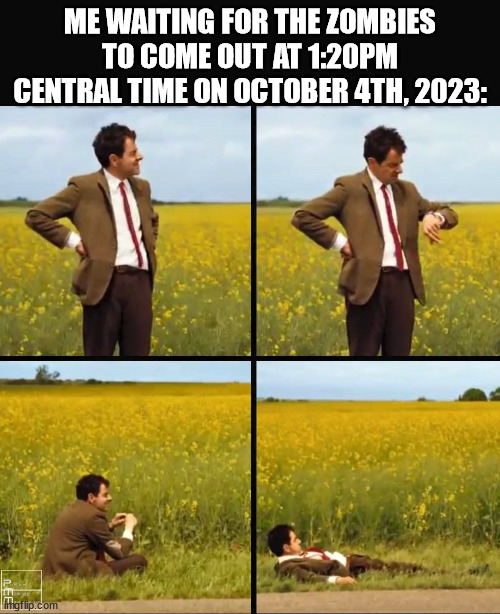This meme features the caption "Me waiting for the zombies to come out at 1:20 p.m. Central Time on October 4th, 2023." It consists of four different images of a man wearing a suit, which includes a brown jacket, a white button-up shirt, a brown tie, and presumably black or brown pants. The setting is an open field with tall weeds under a blue sky. 

In the first image, the man is standing with one hand on his hip, looking away in a direction off-camera, seemingly towards the sky. In the second image, he is glancing down at his watch, appearing to check the time. The third image shows him twiddling his thumbs while looking straight ahead, portraying a sense of boredom or anticipation. The final image depicts the man reclining on the ground, propped up slightly, further emphasizing his wait.